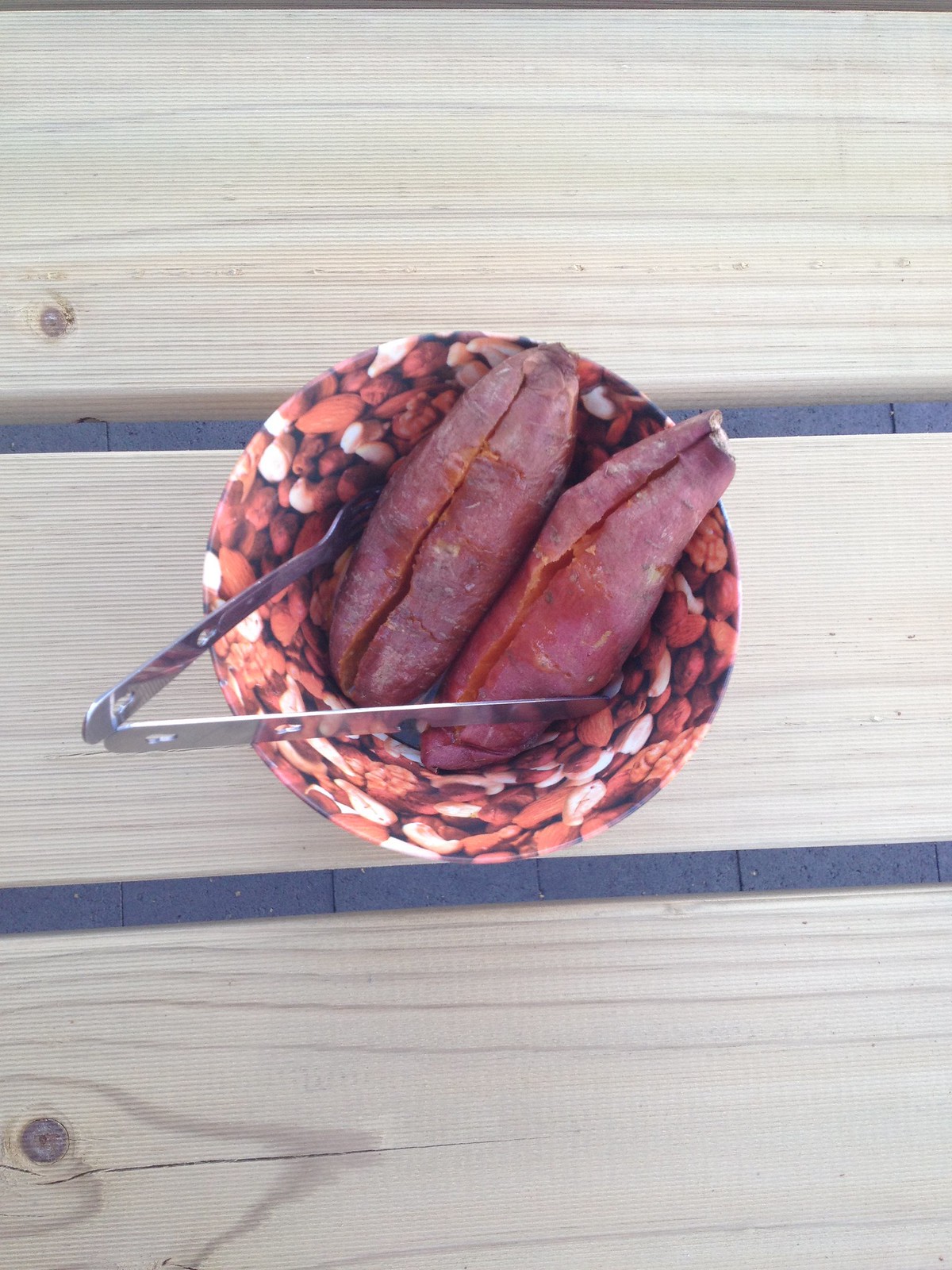This color photograph captures a detailed scene on a light blonde wooden picnic table characterized by visible planks separated by gaps, revealing a gray concrete surface beneath. Central to the image is a bowl adorned with a printed pattern featuring assorted types of nuts and cashews. Inside the bowl rest two brownish-purple tubers, likely sweet potatoes, each with a cut along the center but not split open, leaving the insides hidden. Two utensils, possibly tongs or bent forks, protrude from the left side of the bowl, aiding in holding the tubers. The photograph, taken from a top-down perspective, is notably taller than it is wide. The bottom plank of the table prominently features a knot with a small crack extending downward, adding a rustic charm to this serene and unpopulated setting.